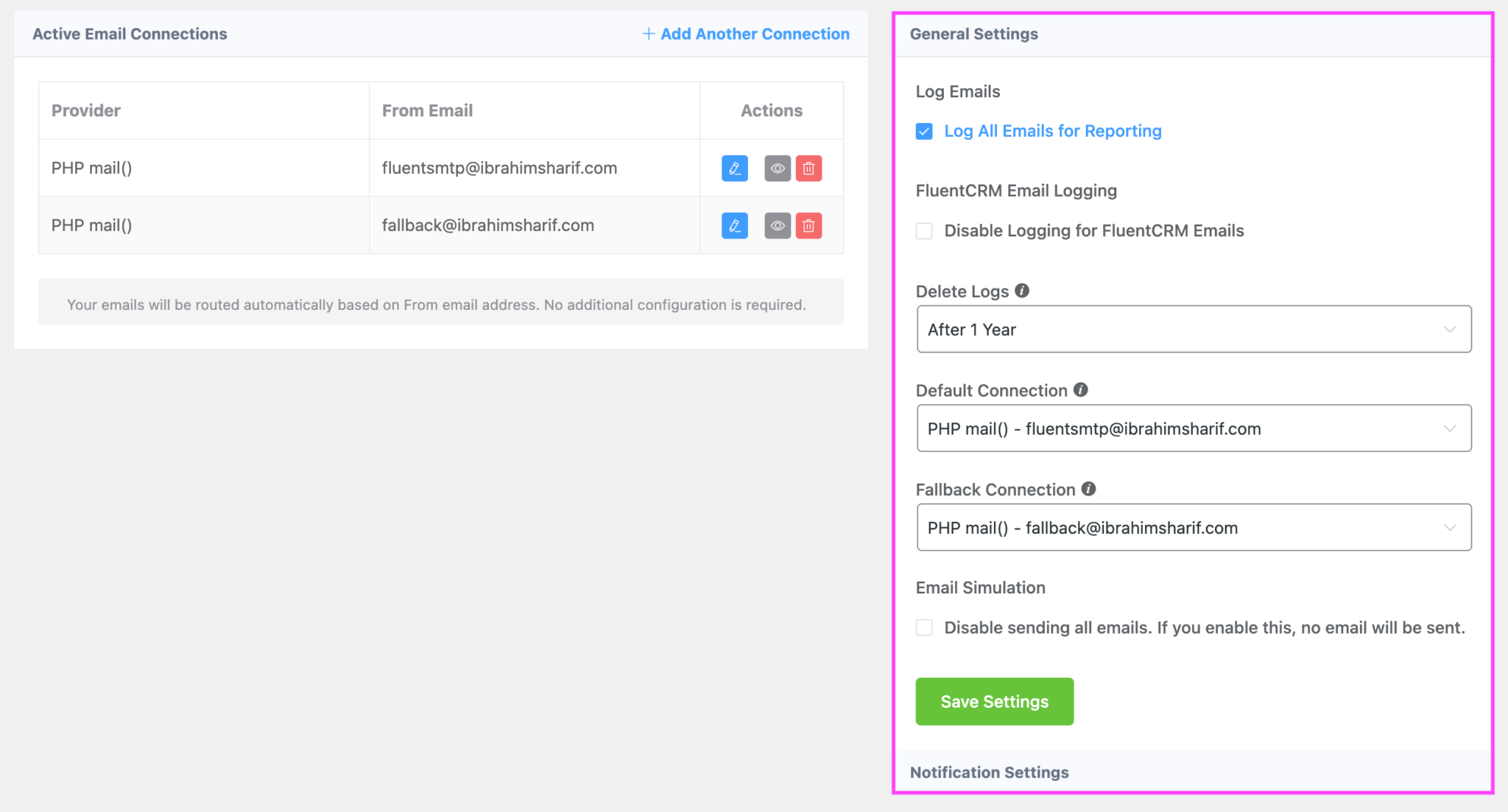This screenshot captures a section of a website interface dedicated to email management. In the top left corner, the heading reads "Active Email Connections." Directly below, there is a table that organizes the data into three columns labeled "Provider," "From Email," and "Actions."

In the "Provider" column, both entries list "PHP Mail." The "From Email" column lists two distinct email addresses: the first one is "fluentSMTP@brahmanhariff.com," and the second is "fallback@brahmanhariff.com." The "Actions" column for each row contains three icons, colored blue, gray, and red, though their specific functions are not clearly visible.

On the right side of the screenshot, there is a prominent settings panel outlined by a thin purple box. Within this panel, there's a section labeled "Log Emails" with a descriptive note "Log all emails for reporting," and the associated checkbox is checked, indicating that email logging is enabled.